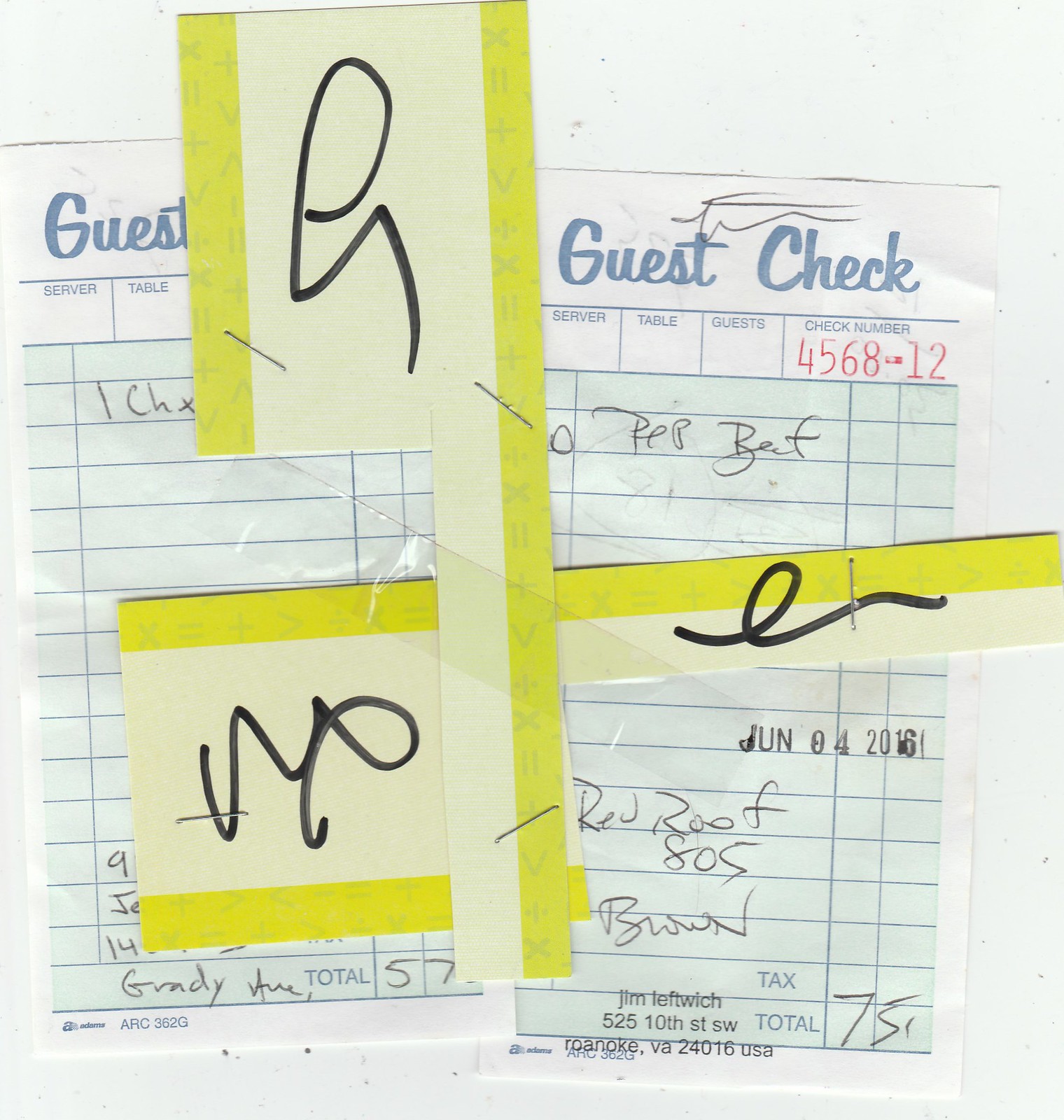This is an overhead photograph of two guest checks from a restaurant. Both checks are light green with a white border, and at the top in blue cursive, they say "Guest Check." Each check features empty boxes for "server," "table," and "guest," but the one on the right has the check number "5484568-12" printed in red. Handwritten in gray pencil on the left check is "1CHX," while the right check reads "PEPBEEF," potentially indicating a roast beef dish. The total on the left check is "$7.50," while the number “570” appears near the bottom, though it's clarified to be "$7.50."

There are yellow and white sticky strips across the checks, held together by four staples. One sticky strip features curly black lines in three spots. Additionally, there is a marking on the left check, "JUN04-0216," possibly a date—June 4, 2016. At the bottom of the right check, it reads "Jim Leftwich, 525 10th Street Southwest, Roanoke, Virginia, 24016, USA." The photo has a predominantly white background, with the checks adding hints of yellow, blue, and green, creating a collage-like appearance. The checks also feature a note directing to "Beadaholique.com for all of your beading supply needs."